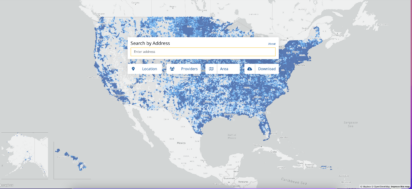The blurred image features a detailed map of the United States, Canada, and Mexico. The majority of the map is covered with blue pinpoints, concentrated primarily in the northeastern United States, with fewer in the western regions. Canada and Mexico appear faded compared to the more prominent United States. Centrally located atop the map of the United States is a search bar that reads "Search by address," although the text is somewhat blurred. Below this search bar, there are several indistinct buttons, one possibly related to location services. The distribution of pinpoints suggests a densely populated or actively targeted region in the upper northeast, tapering as one moves westward.